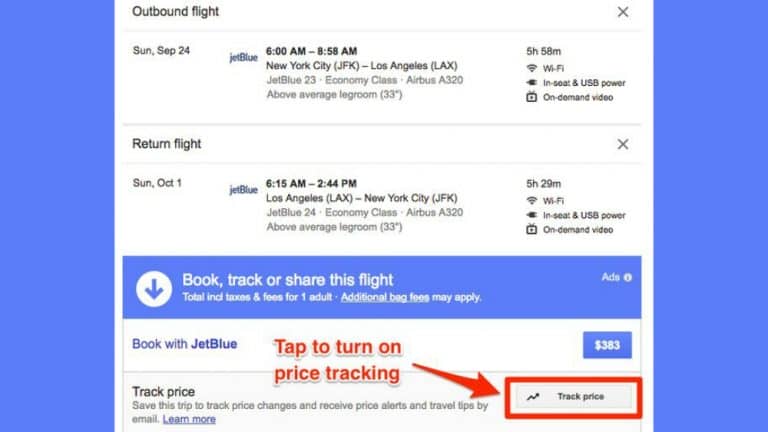### Detailed Descriptive Caption of the Flight Information Screenshot

The screenshot showcases detailed flight information presented against a backdrop of light royal blue vertical rectangles flanking the left and right sides. At the center, a white box houses the key details of the flights, segmented by thin horizontal gray lines that nearly span the width of the box.

#### Outbound Flight Section
At the top-left corner, the text "Outbound Flight" is displayed. In the upper-right corner, a gray "X" icon allows for cancellation. Below it, the flight information is listed in a structured row:
- **Left Column:**
  - **Date:** Sunday, Sep 24
  - **Airline:** JetBlue
  - **Flight Details:** 6:00 a.m. to 8:58 a.m. (New York City JFK to Los Angeles LAX)
  - **Flight Number:** JetBlue 23
  - **Cabin Class:** Economy
  - **Aircraft:** Airbus A320
  - **Additional Info:** Above-average legroom (33 inches, in parentheses)
- **Right Column:**
  - **Duration:** 5 hours 58 minutes
  - **Wi-Fi Availability:** Indicated by a Wi-Fi symbol
  - **Power Options:** Plug-in in-seat and USB power
  - **Entertainment:** On-demand video, indicated by a TV icon

A thin dividing line separates the outbound flight details from the return flight information.

#### Return Flight Section
- **Left Column:**
  - **Date:** Sunday, Oct 1
  - **Airline:** JetBlue
  - **Flight Details:** 6:15 a.m. to 2:44 p.m. (Los Angeles LAX to New York City JFK)
  - **Flight Number:** JetBlue 24
  - **Cabin Class:** Economy
  - **Aircraft:** Airbus A320
  - **Additional Info:** Above-average legroom (33 inches, in parentheses)
- **Right Column:**
  - **Duration:** 5 hours 29 minutes
  - **Wi-Fi Availability:** Indicated by a Wi-Fi symbol
  - **Power Options:** Plug-in in-seat and USB power
  - **Entertainment:** On-demand video, indicated by a TV icon

Above this section, a gray “X” icon in the same row as "Return Flight" allows for cancellation, similar to the outbound flight section.

#### Additional Section
Below the flight details, a section serves as a potential advertisement or extra options area:
- **Background:** Blue
- **Icon:** White circle with a downward-facing arrow in the same blue hue as the background
- **Text:** "Book, Track, or Share This Flight"; "Total includes taxes and fees for one adult. Additional bag fees may apply." 
- **Action Elements:** Info circle to the right

#### Booking and Tracking Section
Two more rows follow:
- **Book with JetBlue:** Price and booking action button
  - **Price:** $383, displayed on a white-text, blue-background button
  - **Annotation:** Bubble text stating "Tap to turn on price tracking"
  - **Annotation Arrow:** Red, angling slightly right, widening as it moves rightward
  - **Highlight:** Red rectangular box around the "Track Price" button, which is gray with the text "Track Price"; the left side of the box features an upward arrow, resembling a stock movement symbol.